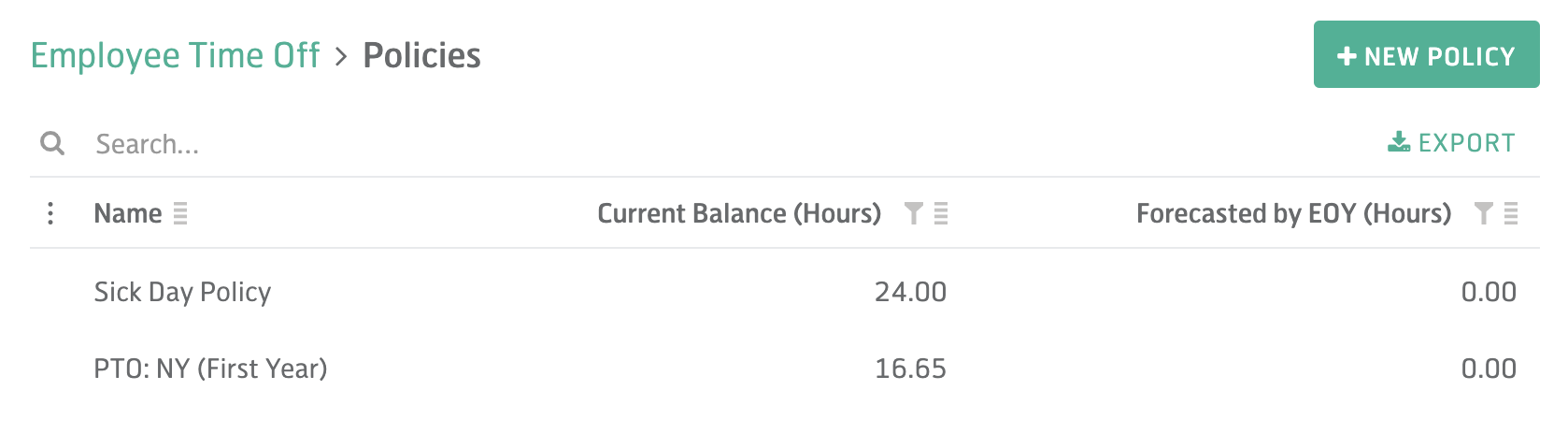The image is a screenshot of a business's sick day policy interface, displayed on a white background. In the upper left corner, the header "Employee Time Off" is written in green. An arrow pointing right leads to the word "Policies" in black. On the far right, there is a green rectangular box containing the text "New Policy" with a plus sign to its left.

Below the header, a magnifying glass icon is positioned next to the word "Search." To its right, there is an export icon followed by the word "Export" in green. Farther down, a left-aligned hamburger menu is followed by the labels "Name," "Current Balance (Hours)," and "Forecasted by EOY (Hours)." To the right of these labels is a second four-bar hamburger menu.

Under the "Current Balance" and "Forecasted by EOY" sections, a radio tower signal icon likely represents forecasted data. Below this, the text reads "Sick Day Policy" followed by "24.00" and "0.00," indicating a current balance of 24 hours and zero hours forecasted by the end of the year. Further down, "PTO: NY first year" has figures "16.65" and "0.00," indicating 16.65 hours of paid time off available in the first year and none forecasted by the year-end.